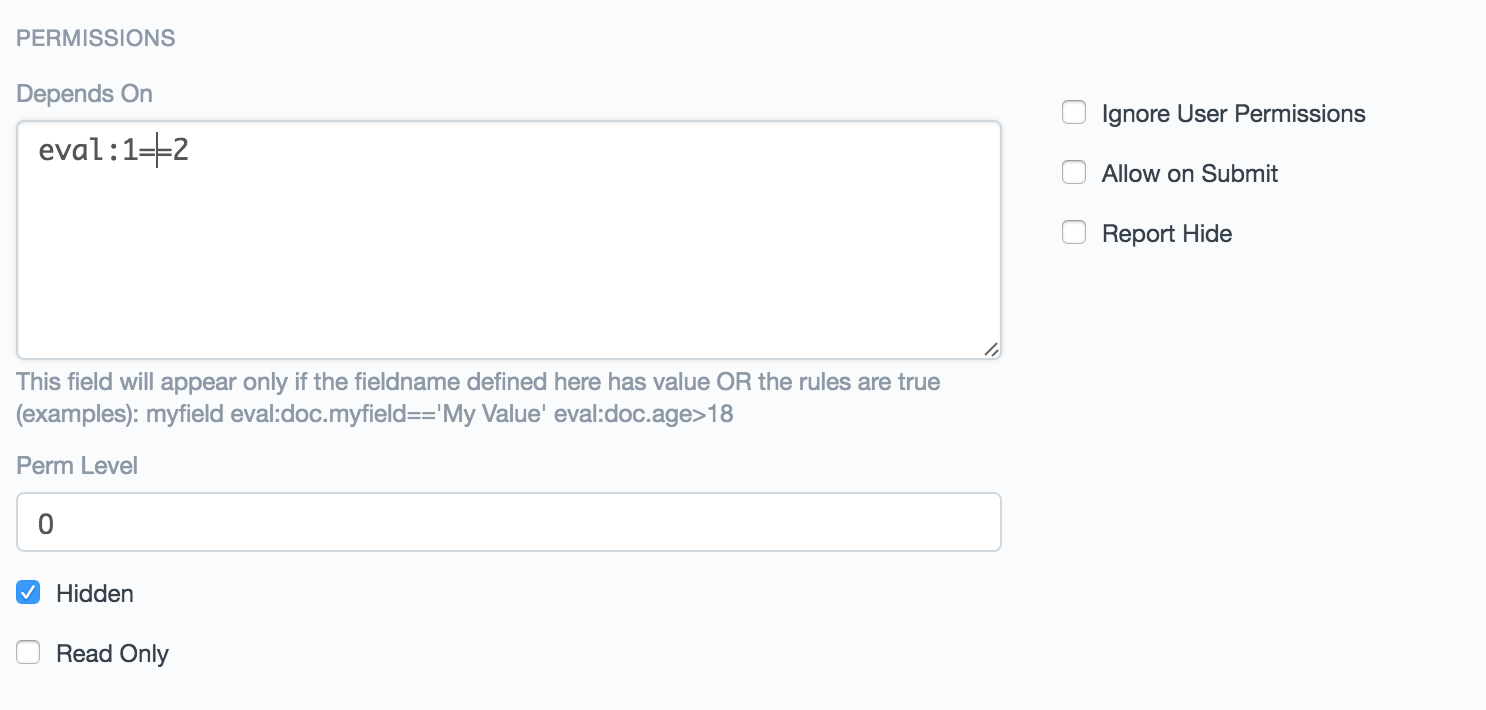The image depicts a gray interface page with several distinctive elements and text fields. At the top, in a slightly darker gray shade, the word "PERMISSIONS" is displayed in all capital letters. Below this header, there is a small section labeled "Depends On," accompanied by a white text box with a thin gray border. Inside this box, black text reads "EVAL: 1 == 2". Notably, there is a black cursor line between the two equal signs.

Underneath this, a paragraph in gray text explains the functionality: "This field will appear only if the field name defined here has value or the rules are true". It provides examples such as "my_field" followed by "eval: doc.my_field == 'my value'" and "eval: doc.age > 18".

Further down, there is a label "Perm Level" with an adjacent white field containing the number "0". Below this, there are two checkbox options: the first one labeled "Hidden" is checked and highlighted in blue, while the second one, labeled "Read-Only," remains unchecked.

To the right side of the interface, there are three additional checkboxes, all of which are empty: "Ignore User Permissions," "Allow on Submit," and "Report Hide."